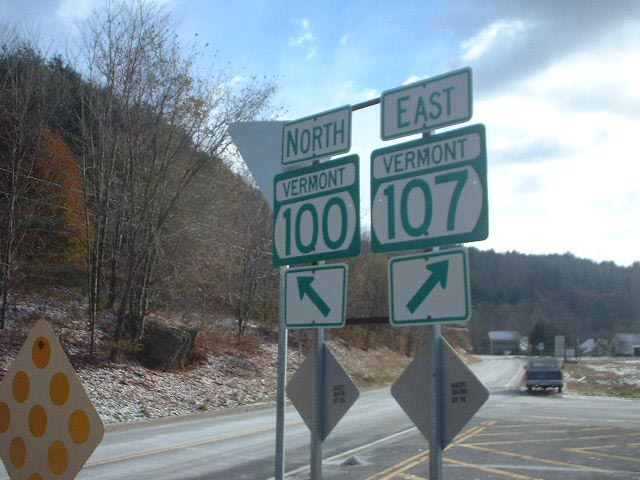This photograph captures a serene rural scene in Vermont, characterized by a cluster of road signs prominently featured in the foreground. The main focal point is a signpost displaying multiple directional signs. The uppermost sign indicates "North Vermont 100" with an arrow pointing diagonally to the left. Adjacent to it, another sign reads "East Vermont 107," directing to the right with a diagonal arrow.

The setting hints at either fall or winter, as suggested by the undulating hills in the background, adorned with trees and brush that may be either bare or changing colors. A pickup truck is stationed on the right-hand side of the image, adding a touch of rustic charm. 

Additionally, in the lower left-hand corner of the photograph, there is an unusual road sign. It is square but positioned like a diamond, featuring nine yellow circles on its surface. This unique sign adds an interesting visual element to the overall composition. All these features come together to create a detailed and picturesque snapshot of rural Vermont.